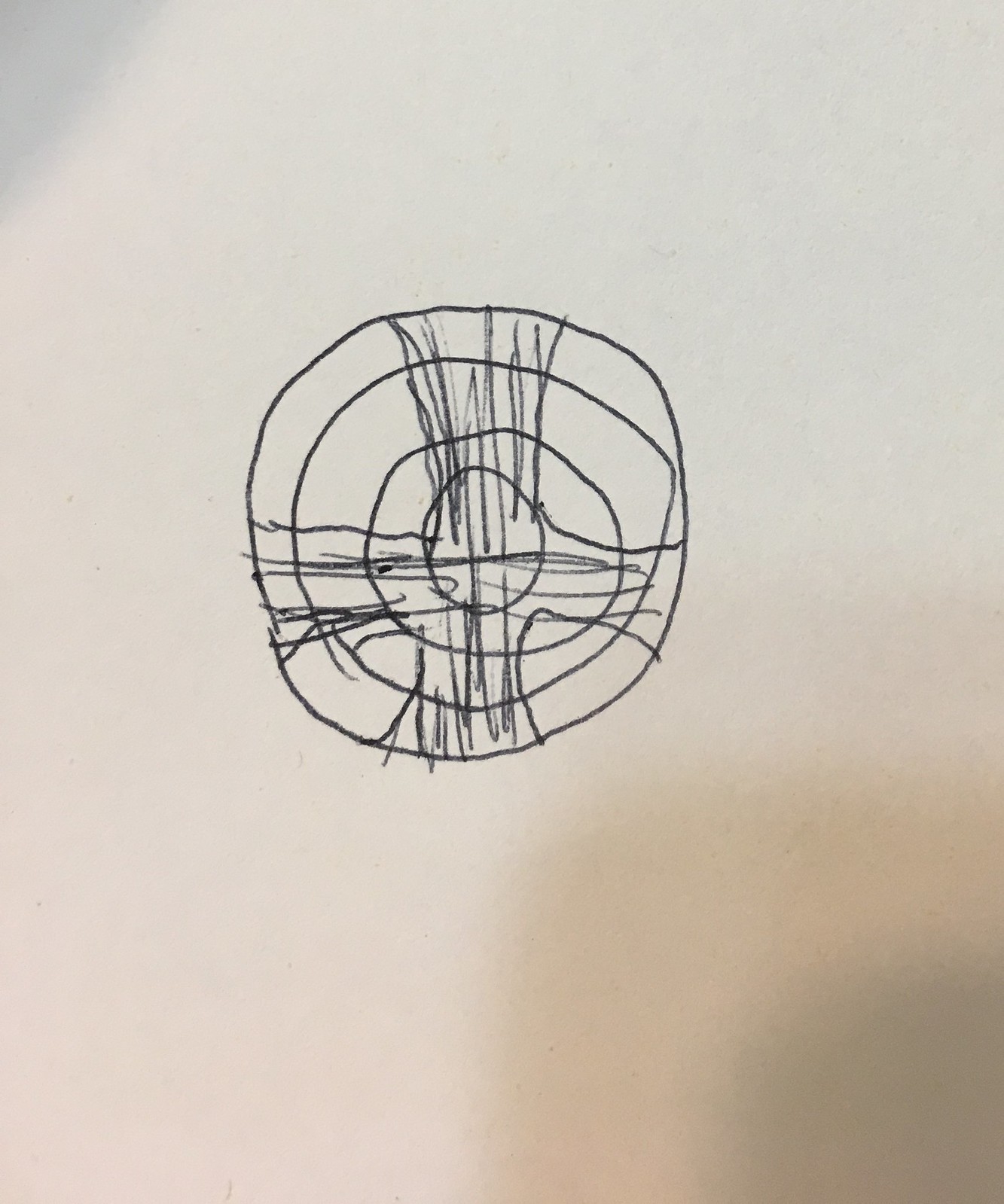A simplistic pen drawing showcases a series of concentric circles, each one nested within the other, culminating in a small central circle. Overlaying these circles is a prominent cross, extended vertically from the top to the bottom and horizontally from the right to the left edges of the largest circle. The intersection of the cross is accentuated by bold, darkened lines, creating a stark contrast against the white background. The entire drawing is rendered on plain white paper, with its amateur quality lending a raw, unrefined charm to the artwork.